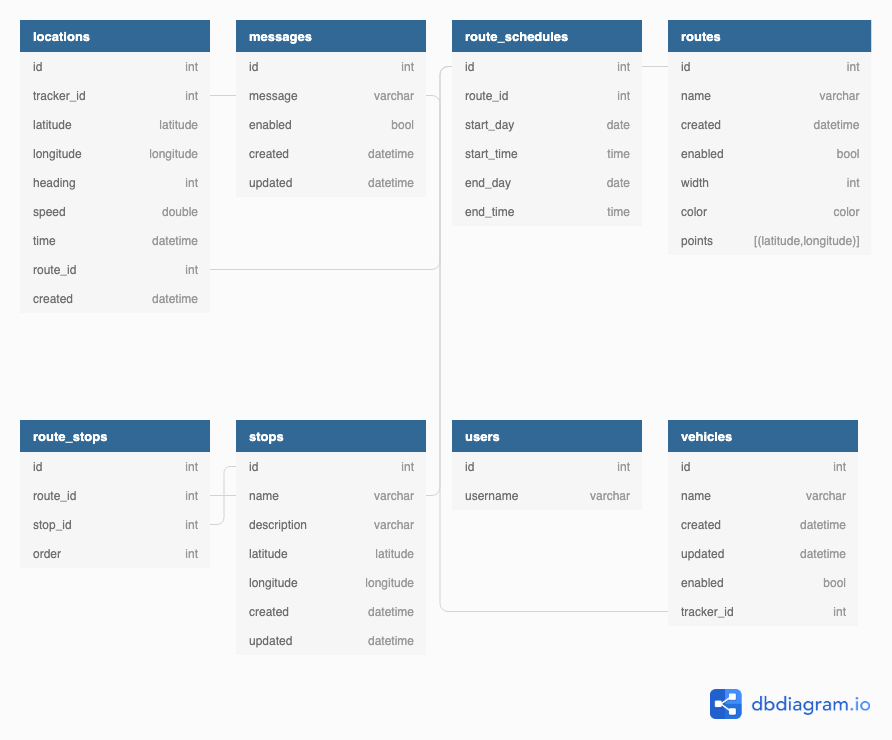This image is a desktop screenshot showcasing a database schema diagram, visually represented with multiple interconnected tables. 

In the top left, a table named "Locations" is highlighted against a predominantly navy background. This table consists of several columns:
- `ID` (Int)
- `Tracker_ID` (Int)
- `Latitude` (Double)
- `Longitude` (Double)
- `Heading` (Int)
- `Speed` (Double)
- `Time` (DateTime)
- `Route_ID` (Int)
- `Created` (DateTime)

Adjacent to the "Locations" table on the right is another table labeled "Messages." This table includes:
- `ID` (Int)
- `Message` (Varchar)
- `Enabled` (Boolean)
- `Created` (DateTime)
- `Updated` (DateTime)

A faint gray line can be seen linking the "Locations" table to the "Messages" table, indicating a relationship between them.

The third column, titled "Route_Schedules," contains:
- `ID` (Int)
- `Route_ID` (Int)
- `Start_Day` (Date)
- `Start_Time` (Time)
- `End_Day` (Date)
- `End_Time` (Time)

This table is also connected by light gray lines to the "Messages" table and the "Locations" table, suggesting relational links among them.

Additionally, the database schema includes five other unspecified columns, indicating a more complex structure not fully detailed in the description.

In the bottom right corner of the image, the name "dbDiagram.io" is displayed in predominantly blue letters next to the company logo, signifying the platform used to generate this schema diagram.